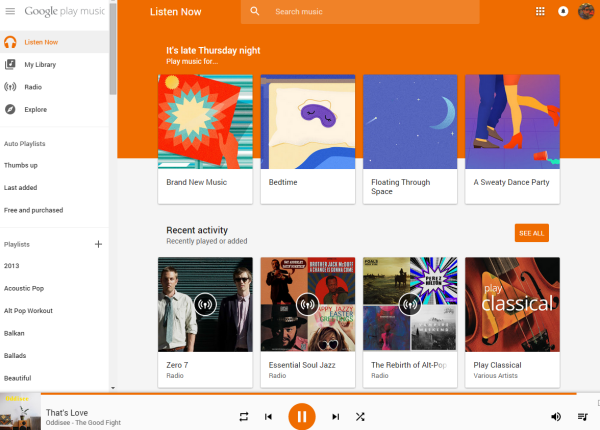The image is a screenshot of a Google Play Music interface on a mobile device or computer. On the left-hand side, a vertical menu displays various options, each with icons and text labels. At the top of the menu, there's an orange headphone icon labeled "Listen Now," followed by a grid-like icon labeled "My Library," an antenna icon labeled "Radio," and a circular icon labeled "Explore." Further down, the menu continues with text-only options, including "Auto Playlist," "Thumbs Up," "Last Added," "Free and Purchased," "Playlist," "2013," "Acoustic Pop," "Alt-Pop Workout," "Balkan," "Ballads," and "Beautiful," suggesting an alphabetical order and that the list continues.

At the top of the interface, the text "Listen Now" is highlighted in orange. Next to it is a search bar for finding music. Below this, the main section of the screen is divided into clickable rectangular tiles. The top row features four sections that can be selected, while the bottom row, under the heading "Recent Activity," shows another set of four selectable tiles. This layout allows users to easily navigate through various music options and recently played content.